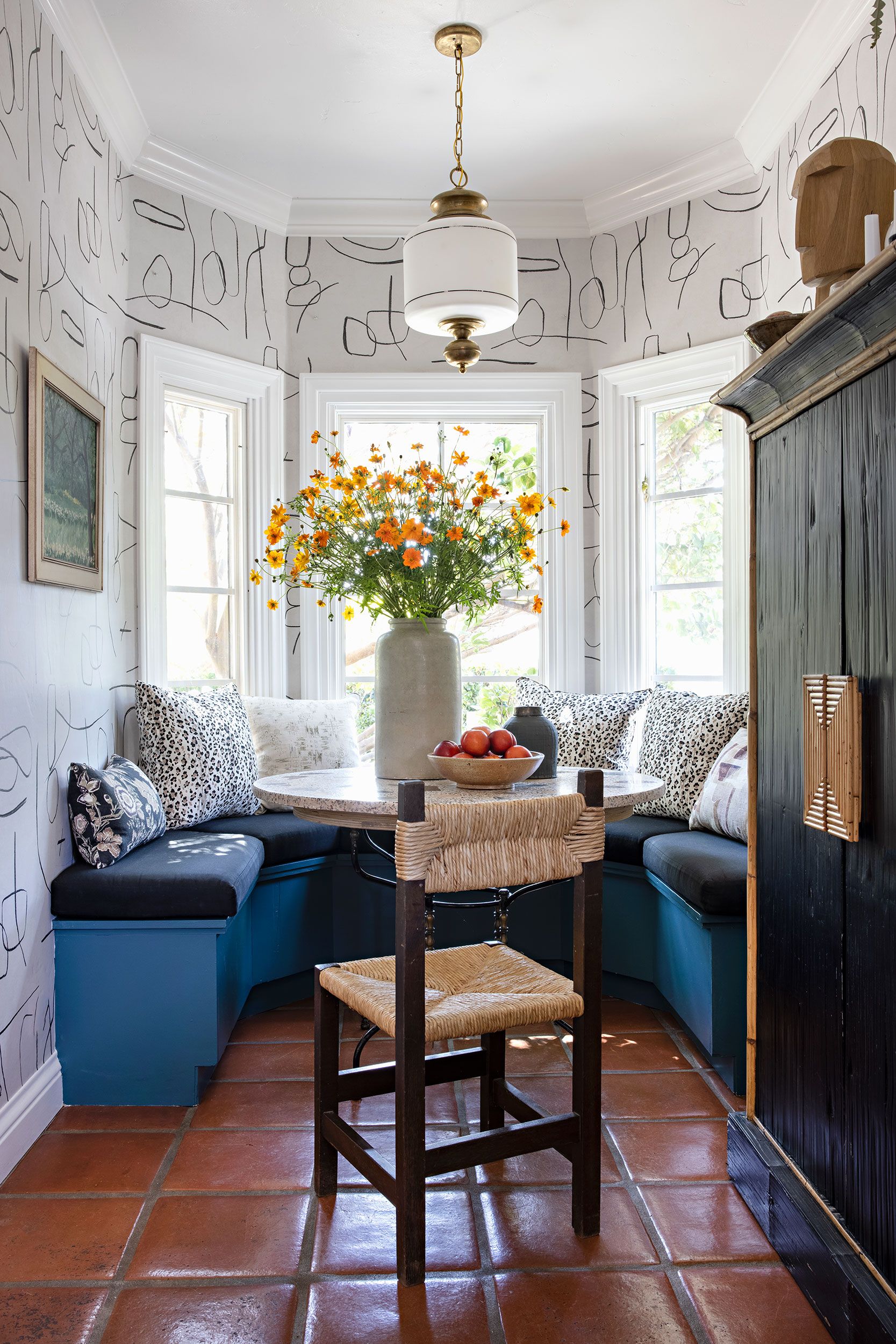The photograph captures an inviting, brightly lit breakfast nook with an array of distinctive features. The room features a dark brown tile floor and a central round marble table. At the center of the room, there’s a brown wooden chair with a wicker backrest and seat. Surrounding the table is a semi-circular blue wooden bench adorned with blue cushions and white and black pillows, providing a cozy seating arrangement. The backdrop consists of three white-framed French windows arranged in an angled, rounded shape, allowing sunlight to pour in. The walls are decorated with light-colored wallpaper, featuring a playful pattern of black lines and circles. A small, golden chandelier with a white glass portion hangs from the ceiling, casting a warm glow over the table. The table itself is embellished with a tall cream-colored vase filled with a vibrant arrangement of orange and yellow flowers and greenery. Next to this, there is a wooden bowl filled with peaches, adding a touch of homely charm to this serene and welcoming space.